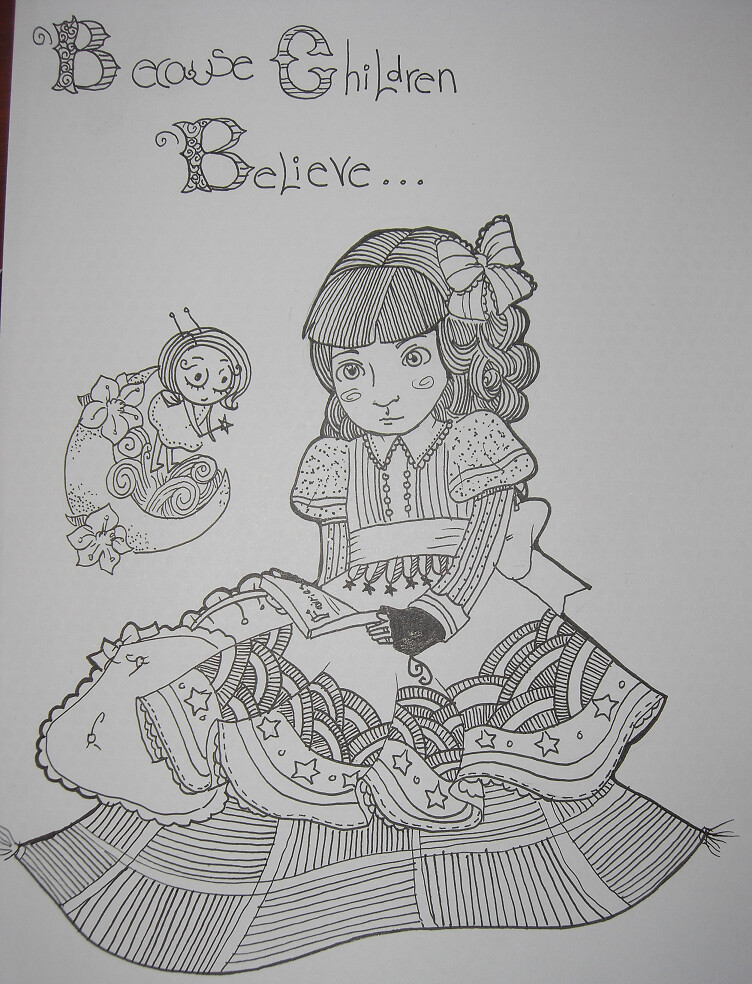This black and white ink drawing captures a whimsical scene featuring a young girl who has a doll-like appearance, dressed in an elaborate, Victorian-style gown adorned with stars and patchwork designs. The girl, who has bangs and curls in her hair, which is complemented by a bow, is engrossed in reading a book. Her dress has elements resembling rainbows or stripes, and she may appear to be wearing black gloves on her left hand or her dress sleeves might just extend over her hands.

To her left, a small fairy with big, circular eyes and a bob hairstyle stands on a crescent moon embellished with flowers. The fairy, who is holding a wand, appears somewhat shocked. Above this enchanting scene is the text "Because Children Believe," with an emphasis on the elegant lettering of the capital letters B, C, and B. The overall composition gives off a magical, dreamy atmosphere, capturing the essence of childhood wonder and imagination.